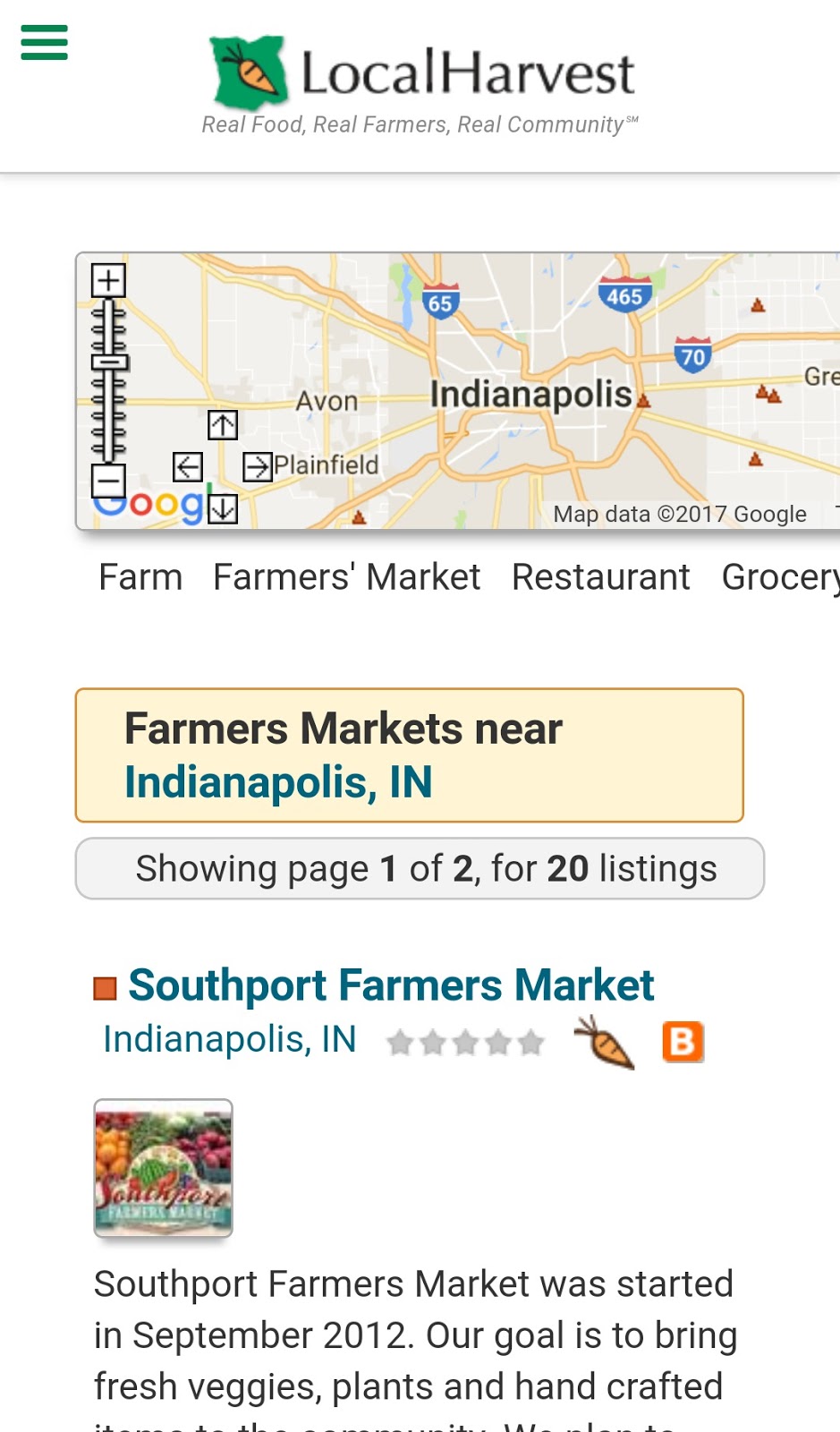This image is a screen capture of a cell phone displaying the Local Harvest website. In the upper left corner, three dark green horizontal bars signify the menu options, while to the right, a wavy green icon with an orange diagonal carrot at the center represents the Local Harvest logo. Adjacent to the logo, the words "Local Harvest" appear in black, followed by the tagline "Real Food, Real Farmers, Real Community."

Directly below the header, a Google Maps section prominently features "Indianapolis" in bold black text at the center. An adjustable vertical scale is positioned on the left side of the map. Beneath the map, a navigational menu lists "Farm," "Farmers Market," "Restaurant," and "Grocery."

A yellow box with a tan outline and bold black letters displays the search query: "Farmers Market near Indianapolis, Indiana" in green. Below this, a gray rectangle indicates the pagination: "Showing page 1 of 2 for 20 listings."

The first and only visible listing is titled "Southport Farmers Market Indianapolis, Indiana" in dark green, accompanied by a red square icon to the left. Five grayed-out stars suggest no current ratings. To the right of the listing is a carrot icon and an orange blogger icon. The listing includes a brief descriptive paragraph and a small food image positioned in the upper left corner.